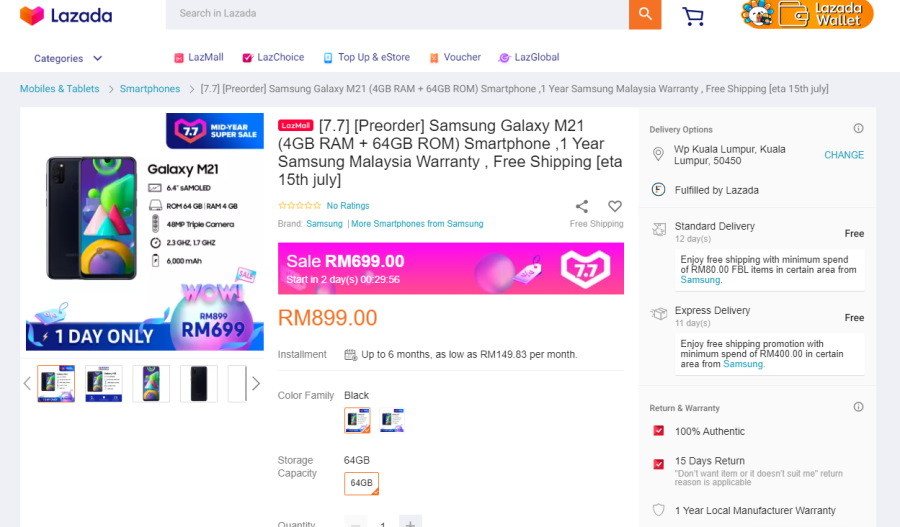The image displays a white-background website, specifically Lazada's homepage. In the top left corner, there's a vibrant logo consisting of an origami-style heart in shades of orange and pink, followed by the name "Lazada." Centered on the page is a light gray search bar paired with an orange search button. On the far right, an "Lazada Wallet" icon is visible, symbolized by a small sun with blue and orange rays.

The main focus of the image below this header is a detailed view of the Samsung Galaxy M21 smartphone. To the left, there is a high-resolution picture of the phone. Just beneath this image is a bright pink banner announcing a sale, offering the phone for RM699.00. Furthermore, below the smartphone's picture, there's a "One Day Only" note, emphasizing the limited-time offer.

On the right-hand side of the phone image, there's a section detailing the order fulfillment information, including the recipient's address. The note indicates that the product is fulfilled by Lazada, with both free standard and express delivery options available.